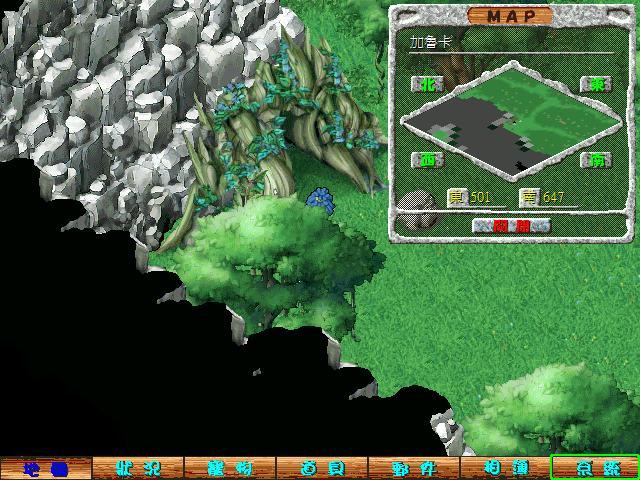This screen capture from a computer game offers an immersive aerial view of a verdant landscape. Dominating the scene, lush green grass stretches widely, interspersed with a few scattered trees. In the top left corner, a rugged hill composed of rough-cut gray stone catches the eye. The hill features an ornate opening embellished with wooden structures and encircled by thriving plant life. The jagged edge of a cliff is visible in the bottom left, adding drama to the terrain.

At the bottom of the screen, a status bar runs horizontally, marked with Asian characters. Additionally, an inset box labeled "map" in the top right corner displays a detailed topographical mini-map. This inset includes cubical symbols and the important numbers 501 and 647, providing critical in-game information.